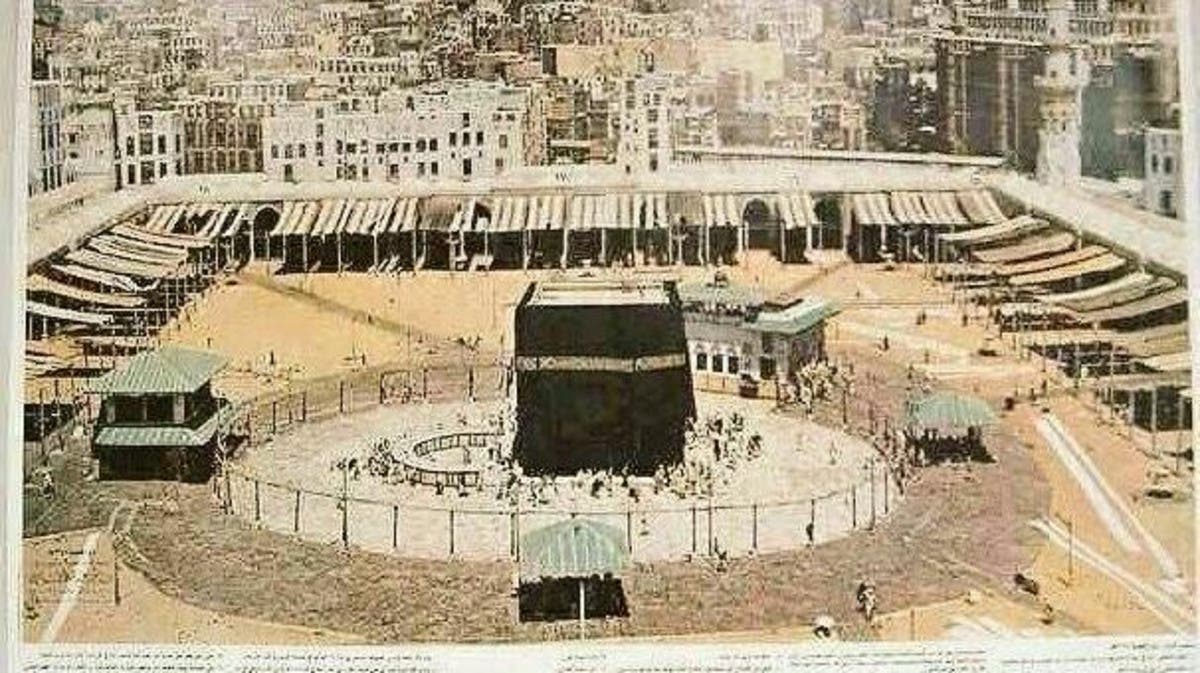This is an old, low-definition color photograph of the Kaaba in Mecca, Saudi Arabia, Islam's holiest site housed within the Masjid al-Haram. The image, likely printed on a yellowing page, depicts a grainy, photorealistic scene under bright, sunny conditions typical of the region. In the center of a circular, sand-covered courtyard stands the Kaaba, a large, dark cubic structure several stories high, encircled by a modest fence. Islamic pilgrims dressed in white are faintly visible, performing the tawaf as they move around the Kaaba. Four smaller buildings are arranged roughly equidistant around this sacred structure, within a wider tan-dirt courtyard bordered by stall-like structures covered with fabric awnings offering shade. The courtyard is framed by an outer building, beyond which looms a cityscape of aged, possibly deteriorating buildings. Two minarets of the mosque are discernible in the background. Some faint Arabic writing is also visible at the bottom of the image, enhancing its historic authenticity.